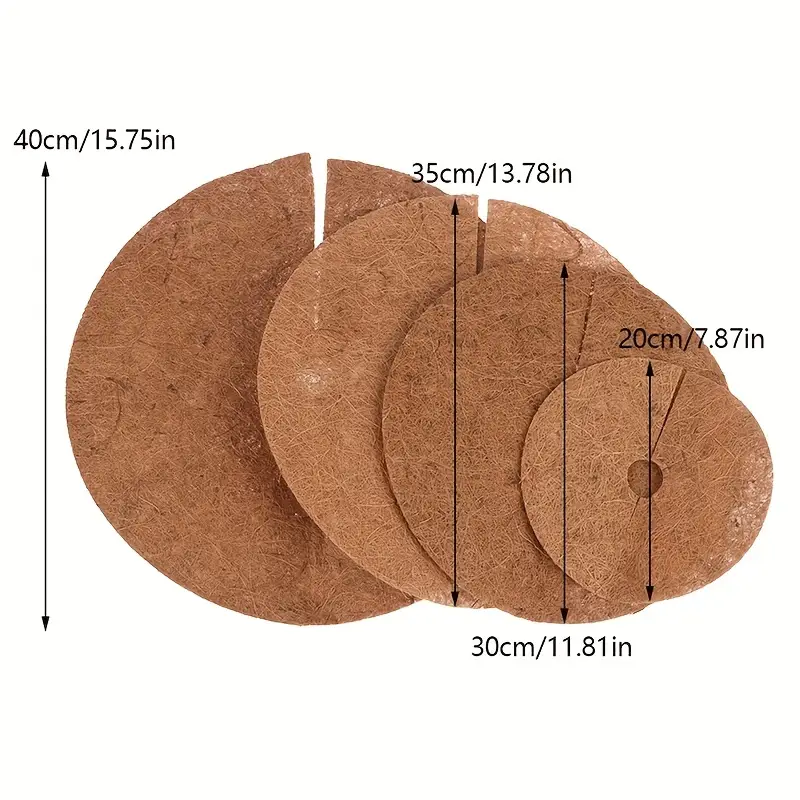The image features a series of four dark brown, circular fabric pieces, arranged in descending size from left to right against a white background, possibly for a store display. Each piece features a small central hole and a slit extending from the edge towards the center, creating an opening that resembles a washer. The sizes of these pieces are clearly marked with measurement lines and black text. The largest piece on the far left measures 40 centimeters (15.75 inches), followed by a piece measuring 35 centimeters (13.78 inches) to its right. Next is a piece measuring 30 centimeters (11.81 inches), and the smallest piece on the far right measures 20 centimeters (7.87 inches). This detailed arrangement and labeling suggest the items are filters or similar products designed to wrap around objects.